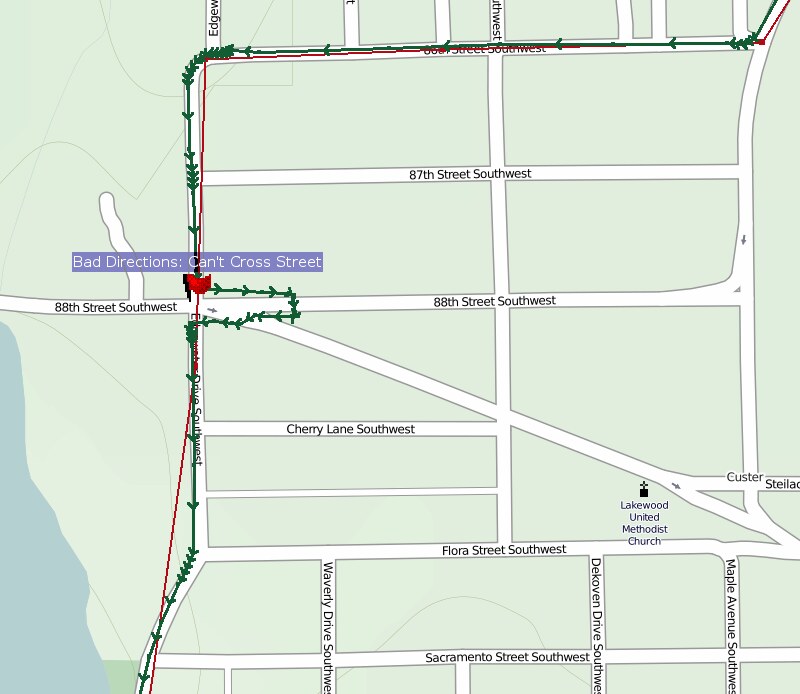In this intricate aerial map, the directions are clearly outlined upon a light gray background, with the lower-left corner distinguished by a blue section, possibly indicating a body of water. The streets are represented as narrow white rectangles, oriented in various directions: horizontal, vertical, and diagonal. At the map's bottom lies Sacramento Street Southwest, flanked by three vertical streets: DeKoven Drive Southwest, Maple Avenue Southwest, and Waverly Drive Southwest. Above, Flora Street Southwest stretches horizontally across the map, intersected by an unnamed vertical road, alongside Cherry Lane Southwest branching off to the left. Further up, the streets are ordered horizontally as 88th Street Southwest and 87th Street Southwest. Notably, on the far left, a road meanders and curves to the right, adorned with a green vine and red line, culminating at the top-right corner. An icon marks the presence of Lakewood United Methodist Church, offering a recognizable landmark within this well-drafted schematic.